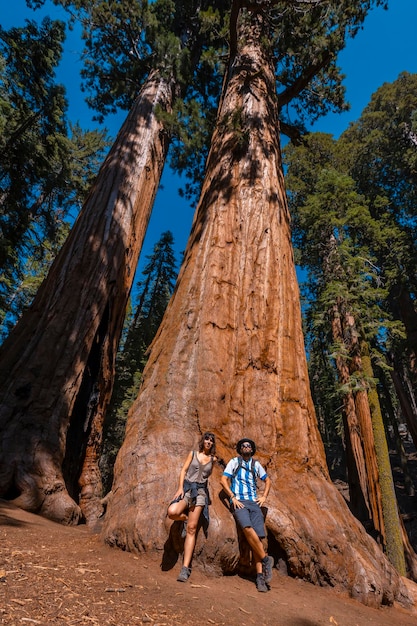In this captivating image, a man and a woman stand side by side, leaning against an enormous sequoia tree, which dominates the scene with its immense height and girth. The towering tree has a reddish-brown, layered bark that transitions to verdant greenery at its upper reaches. The photograph is taken from a low angle, intensifying the impression of the tree's colossal size. The backdrop of a bright blue sky contrasts vividly with the dark brown soil scattered with fallen bark and debris. The male figure, positioned on the right, wears a blue and white striped T-shirt, blue shorts, tennis shoes, and sunglasses. He is bearded, with long hair to his ears, and adopts a hands-on-hips stance. The female figure stands on the left, dressed in a gray tank top, olive-colored shorts, and a sweater tied around her waist. With wavy, shoulder-length brown hair and gray hiking boots, she strikes a relaxed pose with her right knee bent. Together, they appear minuscule next to the giant sequoia, akin to ants dwarfed by a monumental natural marvel.